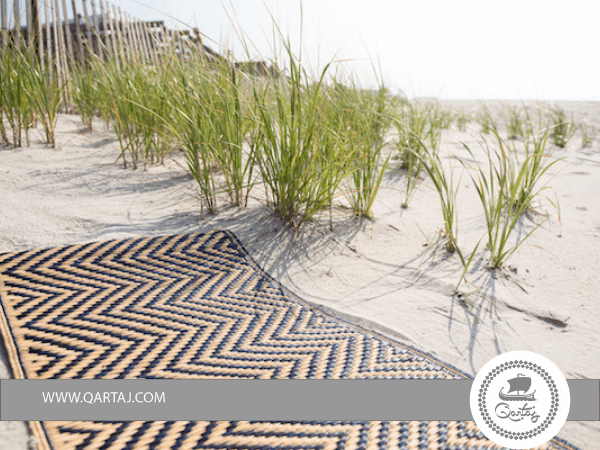The image captures a sunlit beach scene dominated by fine white sand dotted with short, sparse grass. At the background, towards the top left, stands a wooden stick fence, a common sight on beaches. Centered prominently on the sandy terrain is a brown mat with intricate black patterns forming V or M shapes, bordered by a black line. An essential detail is the grey banner running along the very bottom of the image, reading "www.qartaj.com" in white text on the left side, accompanied by a white circular logo on the right. This logo includes a grey silhouette of a ship encircled by two concentric grey circles. The sky overhead appears clear, with the bright daylight illuminating the scene, suggesting a pleasant day at the beach.